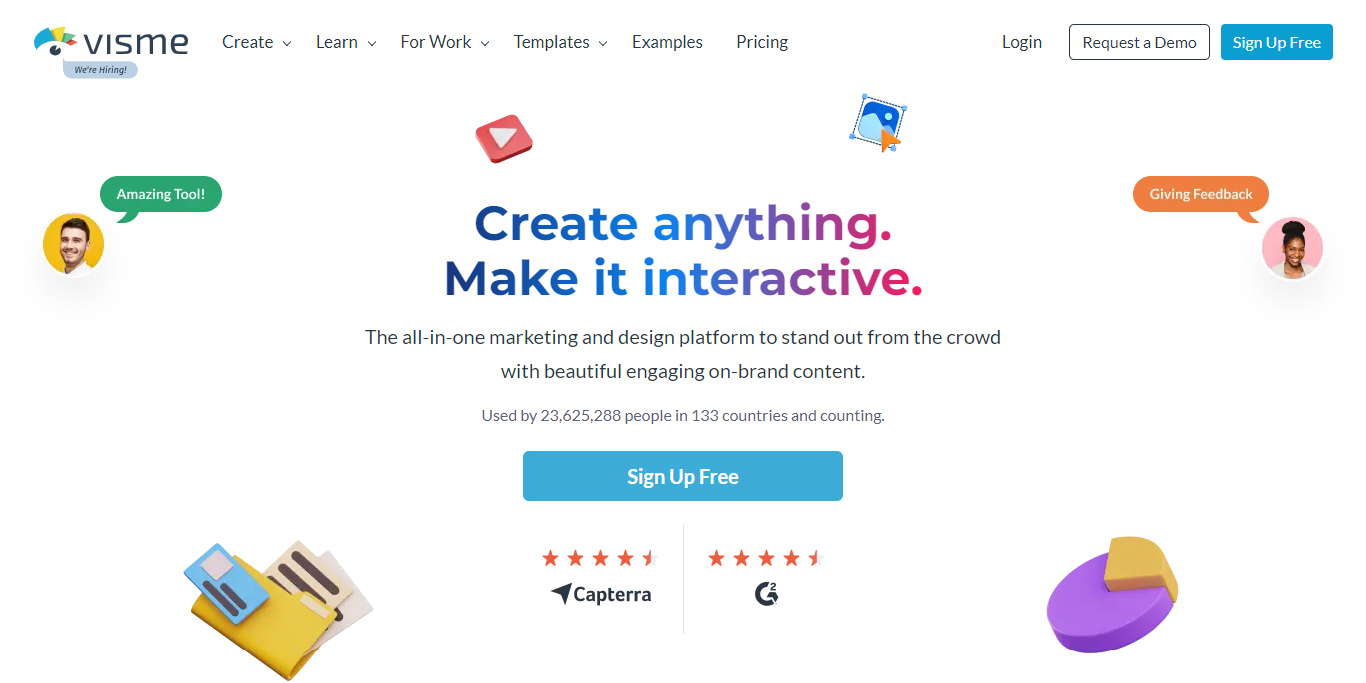The web page features a clean, white background with the brand name "VISME" prominently displayed in the upper left corner. The text is uniform in size and styled in a modern, bubbly yet digital black font. Accompanying the text is a distinctive icon resembling an eye. The eye has a black pupil with a white reflective spot on the upper right, and its "eyelashes" are a series of colorful petals in teal, yellow, green, and pink hues.

Beneath the logo, a gray speech bubble icon states "We're hiring." To the right, the navigation menu is displayed in a light gray font. The menu items include "Create" (with a dropdown arrow), "Learn for Work" (with a dropdown arrow), "Templates" (with a dropdown arrow), "Examples," and "Pricing." Further to the right, options for "Login" and "Request a Demo" are shown. "Request a Demo" appears within a white, dark gray-outlined rectangular icon, while "Sign Up for Free" is presented in a blue background icon with white text.

Centrally, a striking headline reads "Create Anything. Make it Interactive." and features a gradient from dark blue to light blue, transitioning to purple and pink. Below this, a smaller black font declares the platform's value proposition: "The All-in-1 Marketing and Design Platform to stand out from the crowd with beautiful, engaging on-brand content." Finally, in smaller gray text, it notes: "Used by 23,625,288 people in 133 countries and counting."